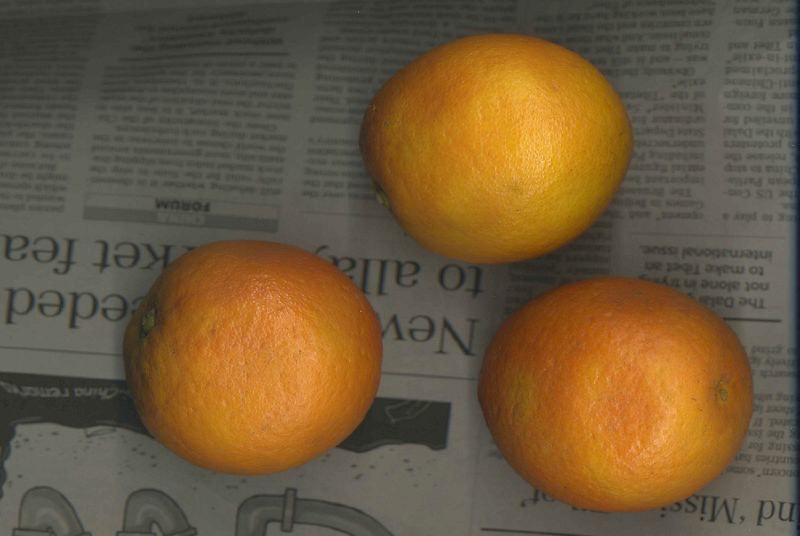This color photograph captures an overhead view of three unpeeled oranges arranged in a triangular pattern on an upside-down newspaper. The image is relatively low in light, casting shadows across the scene and giving the newspaper a grayed, low-contrast appearance. The oranges vary in ripeness and color, with the lower left one being the darkest and most ripe, showing slight dimples and a pinkish cast, which might hint at it being a grapefruit. The bottom right orange, slightly lighter in shade, also shows a stem, and the top center orange is the palest and most uniformly colored, with a reflection of light on its right side. The newspaper serves as a backdrop, its upside-down text and images mostly blurry and unreadable, although discernible words like "NEW" and snippets of headlines hint at economic news. The black font on a white background accentuates the classic appearance of a printed newspaper beneath the bright, organic presence of the fruit.